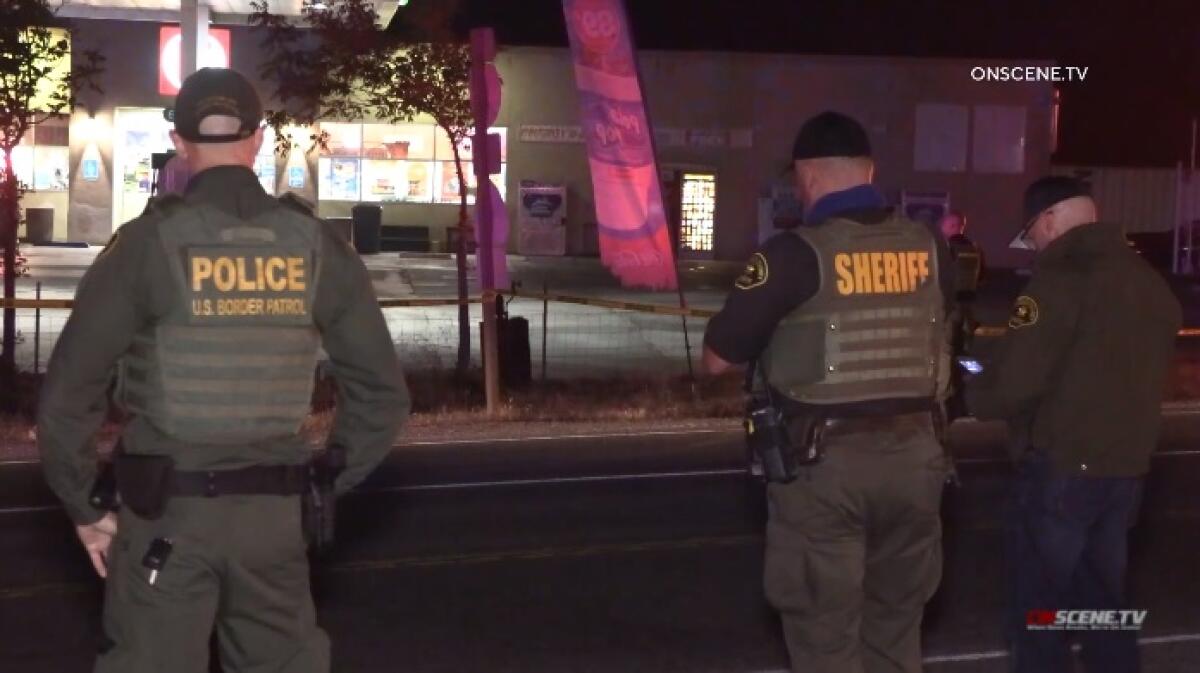The nighttime image, likely a still from a TV program as indicated by the "OnScene.TV" text in white at the top right and the stylized "OnScene.TV" logo at the bottom right, features a trio of law enforcement officers viewed from behind. All are standing along an access road, just behind a guardrail, with a convenience store—potentially a Circle K, identifiable by illuminated advertisements—situated in the background. From the left, the first officer is partially visible, dressed in a green uniform with a black utility belt and a pair of keys hanging over his back pocket. His ballistic vest has 'POLICE' in bold yellow letters and 'U.S. BORDER PATROL' underneath. He wears a black baseball cap. The second officer, towards the right, dons a green tactical vest labeled 'SHERIFF' in yellow, along with green trousers and navy short sleeves. He also sports a black baseball cap and has a walkie-talkie attached to his utility belt. To the far right stands the third officer, clad in a dark jacket with an indiscernible yellow emblem on his left arm and dark navy trousers. He appears to be engrossed in a device with a screen. The three officers, all facing away from the camera, are distinct in their uniforms, yet unified in their stance, possibly indicating a collaborative operation. The backdrop includes a series of windows and lights from the convenience store, a vending machine, fencing, and small trees, adding to the scene's depth and context.